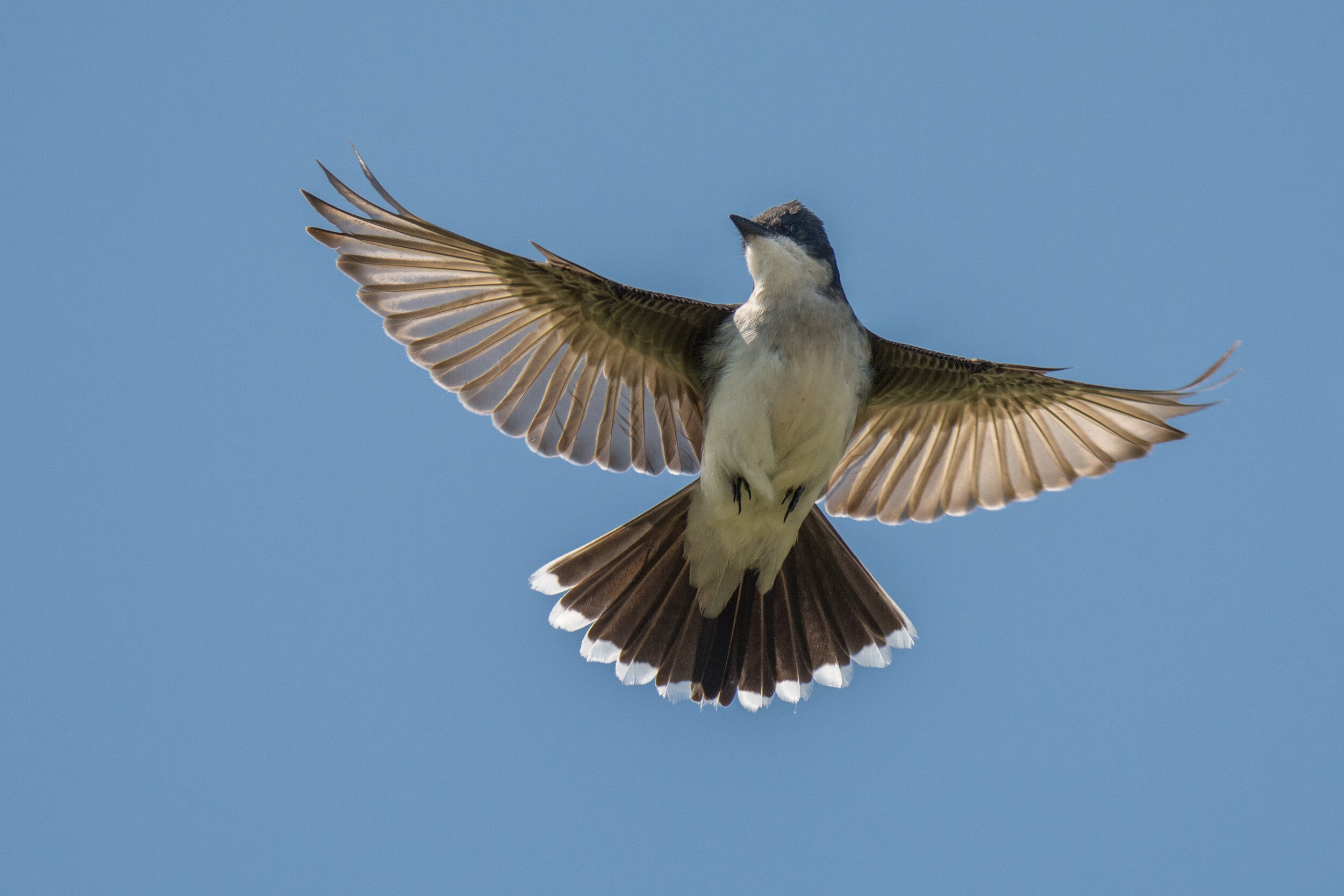The image depicts a majestic bird soaring against a light blue sky with hints of hazy cloud cover. Captured from below, the viewer is presented with a full view of the bird's underside, showcasing its impressive wingspan. The bird's wings are outstretched wide, with feathers that transition from a greenish-gray near the body to translucent white at the tips, arrayed almost geometrically. Its tail feathers splay outwards, primarily brown with white tips. The bird's breast and the lower part of its neck are a fluffy, tufted white. The bottom of its face is also white, contrasting with the top of its head which is a dark color, bordered by its dark beak. The bird’s small black feet are tucked in as it glides gracefully through the sky. The overall look of the image evokes the somber, respectful tone often seen in memorial cards, adding to the dignified and peaceful aura of the scene.